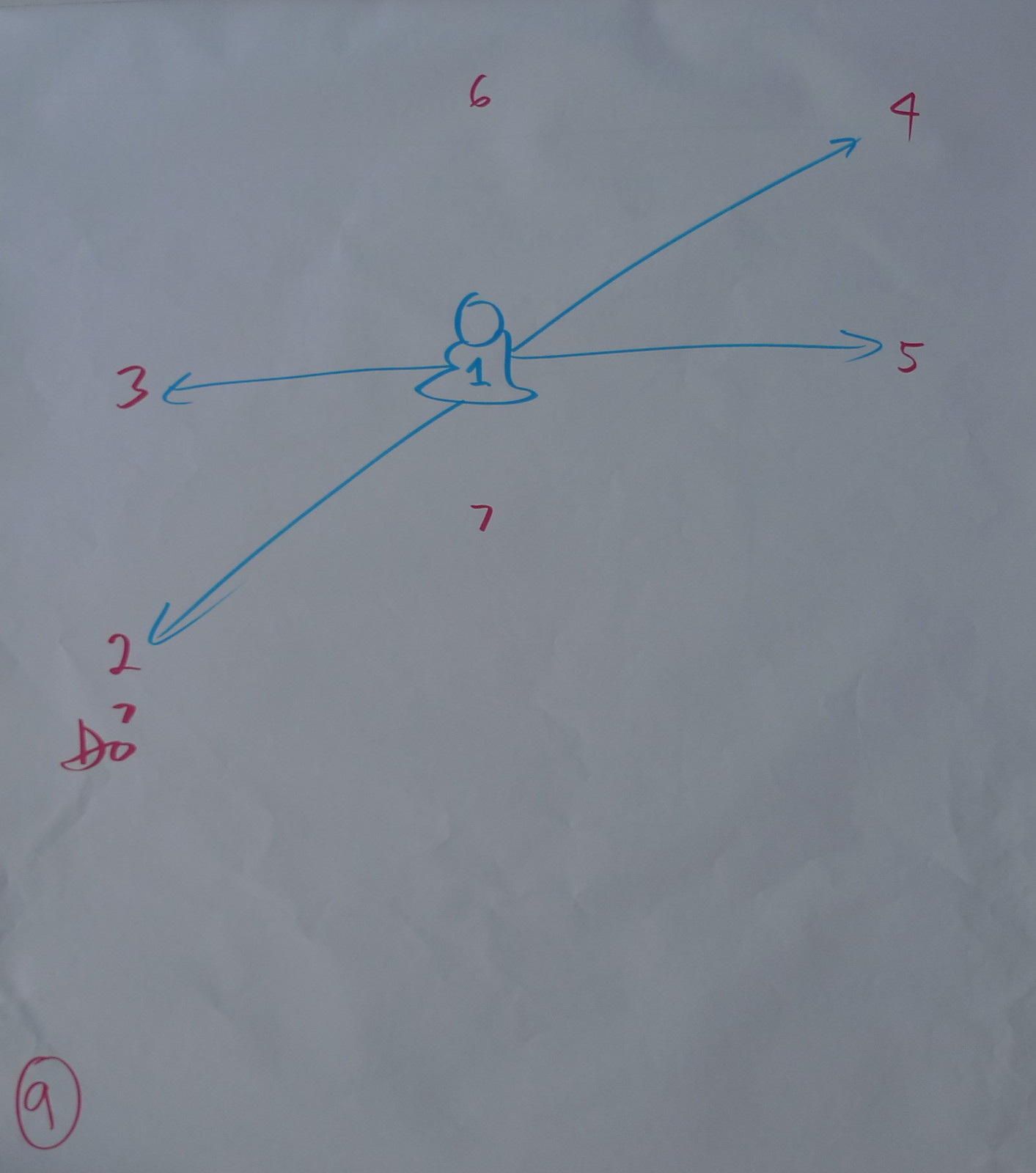The image features a hand-drawn sketch on gray computer paper, marked with various colored numbers and symbols. In the bottom right corner, there's a red number "9" encircled in red. At the top center of the paper, a red number "6" is prominently displayed. Moving to the top right corner, there's a red number "4," with a red number "5" directly beneath it. Also directly beneath the number "6" at the top, you find a red number "7." Toward the top left, slightly down from the center, a red number "2" appears with another red number "7" positioned below it. Additionally, near this area is a red D-shaped figure. Directly horizontal from the red number "5" is a red number "3."

At the center of the paper, a distinctive blue figure stands out, characterized by a circular head and a squiggly, bell-shaped body. This figure features a blue number "1." Four blue arrows emanate from this central figure, each pointing towards different numbers: an arrow towards the red number "3," another towards the red number "2," a third one pointing at the red number "4," and the final one directed at the red number "5."